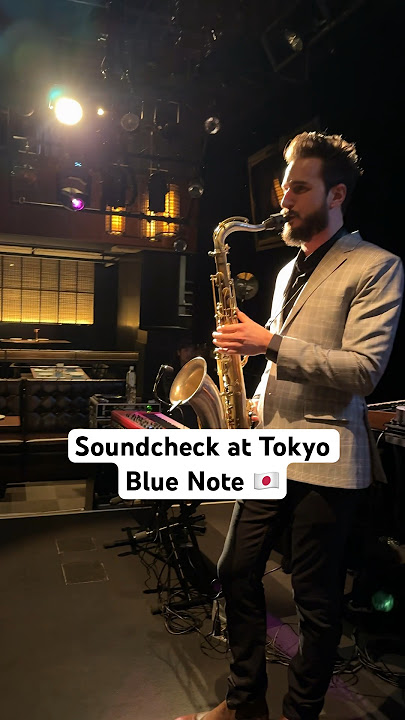A bearded man with gelled or spiked-up hair stands alone on a dimly lit indoor stage, deeply immersed in playing a saxophone. His left hand grips the center of the instrument while the mouthpiece is secured in his mouth. He wears a light gray coat with a slight checkered pattern over a dark shirt, complemented by dark pants and brown shoes. The stage floor is brown, and a spotlight from the upper left corner casts a bright beam on him, highlighting his presence against the otherwise dark backdrop. In the background, there's a red keyboard on the right side and some digital music equipment to the left center, as well as a closed window with a yellow shade. Above the stage, light rigging and a balcony with a railing can be faintly seen. Overlaying the image are black letters on a white background that read "Soundcheck at Tokyo Blue Note," accompanied by an emoji of the Japanese flag.